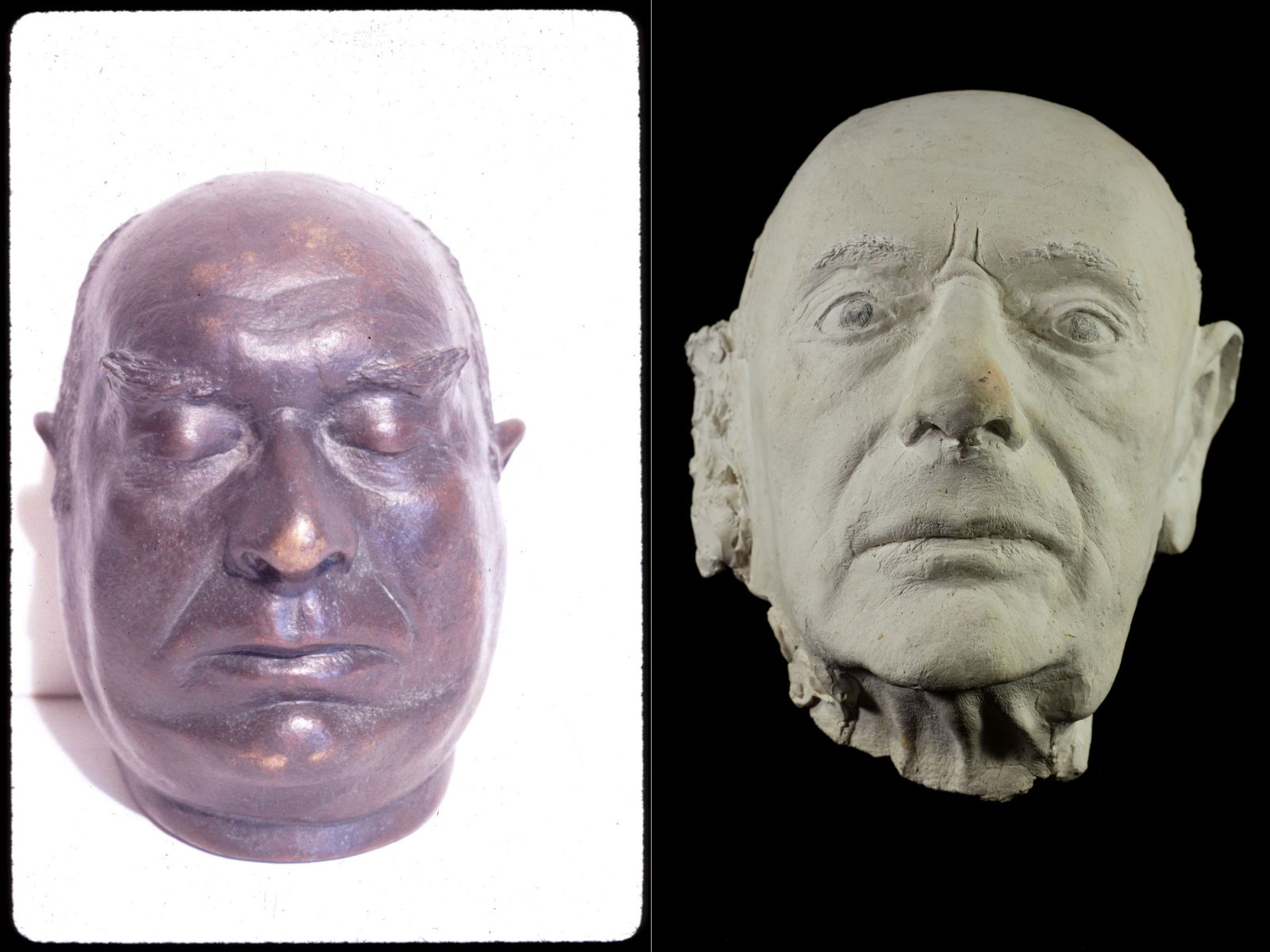This image features a side-by-side comparison of two head sculptures set against contrasting backgrounds. On the left, a bronze statue of a bald man has closed eyes and upward-angled thick eyebrows, giving him a serene or somber expression. His lips are shut tight, and the tops of his ears are just visible against a stark white background. On the right, a partially completed clay portrait depicts another bald man with bright, open eyes and normal eyebrows. His mouth is also closed, and his unfinished ears are still covered in plaster, especially noticeable around the ear area. The clay sculpture has prominent wrinkles running down from his brow and a noticeable piece of clay at the corner of his eye. His nose is marked by a yellow streak, and the background is black, emphasizing the work-in-progress nature of this piece.